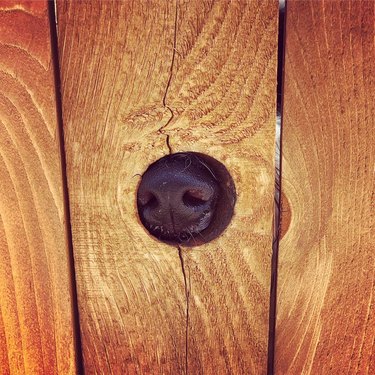The image depicts three vertically arranged wooden slats of varying visibility, with the central slat being fully visible while the left and right slats are partially shown. The wood of the slats is characterized by a textured, medium brown finish with light and dark swirls and markings. A notable feature is a vertically oriented fine slit that runs through the center of the middle slat, which interrupts at a circular hole. This hole perfectly accommodates a large, black dog’s nose, displaying two distinct nostrils. Around the protruding nose, wisps of white fur are visible, suggesting the presence of the dog's snout peeking through. The arrangement of elements, along with the subtle hints of the dog's white fur behind the wooden slats, adds a layer of intrigue to the simple yet charming scene.